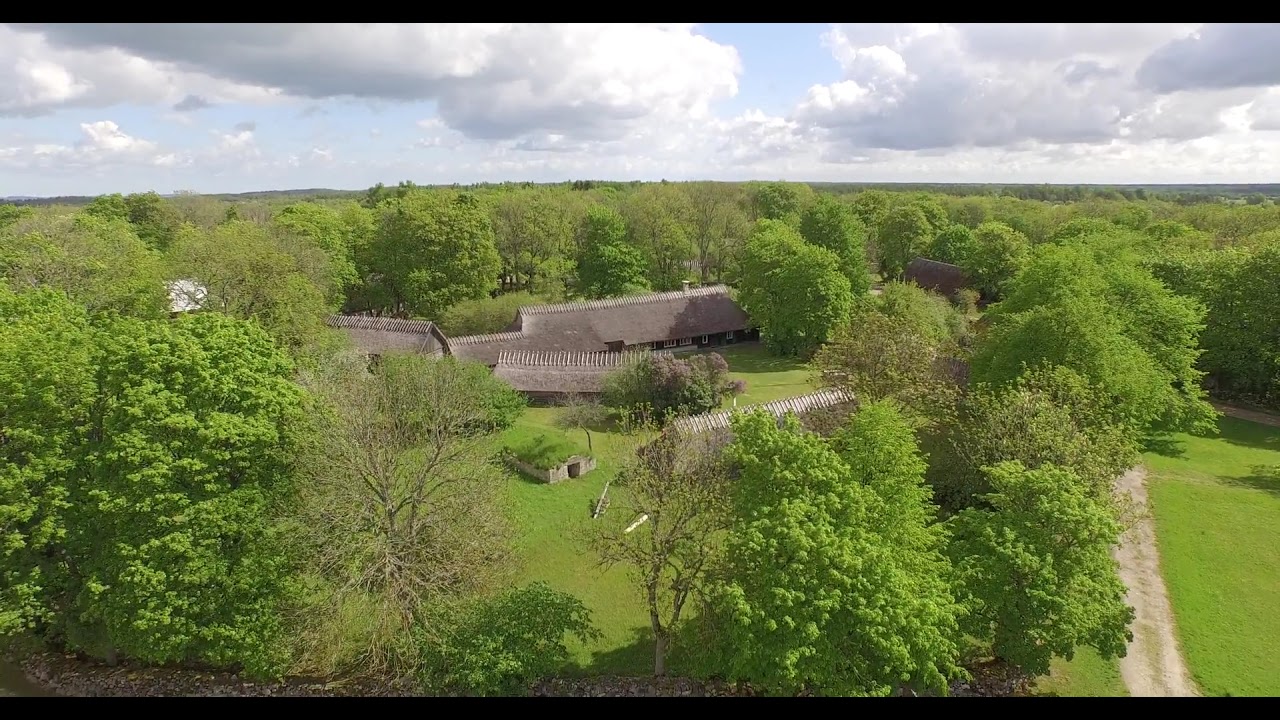The image is an aerial view taken from a high vantage point, possibly a drone, capturing a sprawling agricultural landscape. The panorama showcases a lush, green area dominated by thick clusters of trees and bushes with patches of green grass. The landscape is relatively flat, with no significant hills visible. Towards the lower right-hand side of the image, a dirt road is noticeable, curving through the vegetation. 

In the middle of the scene, a cluster of buildings is prominently visible. A large house with a beige roof and dark-colored siding framed by white windows lies at the center. Beside it, there is a smaller outbuilding made of concrete with an open square door, and a shed closer to the viewer. A gravel driveway, gray in color with a bit of grass growing in the center, stretches from the front towards the back on the left side of the image, branching out toward the house.

The photo is set in landscape orientation, framed by horizontal black strips at the top and bottom, emphasizing the flatness of the terrain and the vastness of the sky above. The sky, occupying the upper fifth of the image, is relatively cloudy with just hints of blue peeking through. The scene, captured in a realistic style, offers a detailed and immersive view of the tranquil agricultural setting.